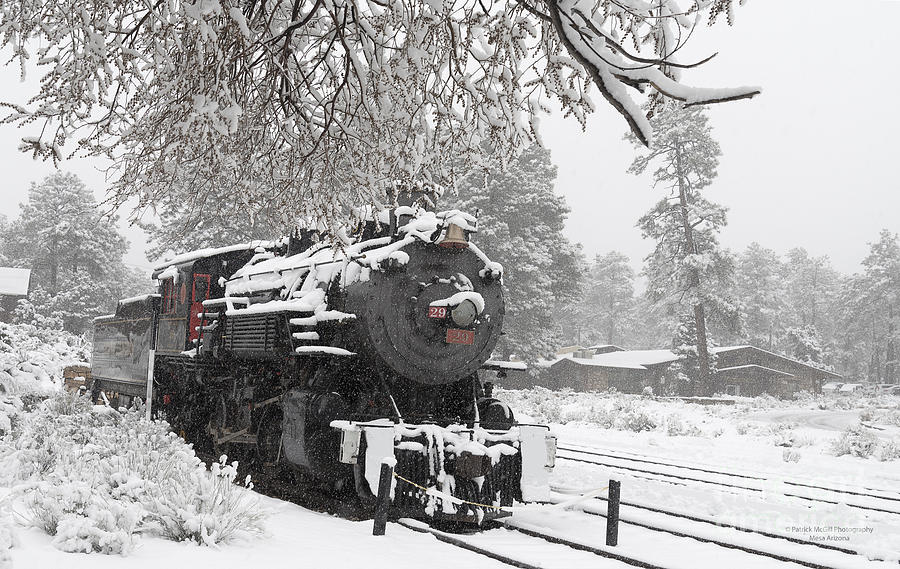In this photograph by Patrick McGiff Photography from Mesa, Arizona, we see an old, decommissioned steam train covered in snow, stationed on snow-covered tracks in the midst of winter. The train, predominantly grey and black with a blanket of white snow on top, stands virtually in the center of the image, indicating it is not in motion. A small rope barrier and markings in front of it suggest it is a preserved exhibit rather than an operational locomotive. 

Surrounding the train are various elements of a cold, snowy landscape. To the left in the foreground, a shrubbery is also cloaked in snow, and tree branches hang into the frame from above. Behind the train, on the right, there are low-lying bungalow-style buildings or lodges with snow-covered rooftops. Dominating their snowy backdrop are tall, snow-laden trees that fade into a blurry, distant forest. The entire scene is under an overcast sky with grey clouds, enhancing the chilled, tranquil atmosphere of this winter wonderland.